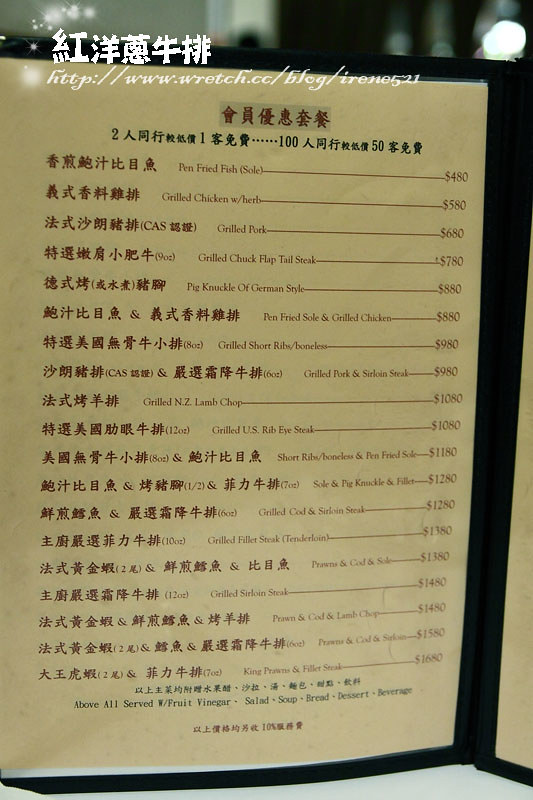The image features a page from a Chinese menu printed on brown paper. Dominating the top of the page, there is some Chinese text with a URL that reads www.rich.cc/blog/Irene521. The menu items are predominantly in Chinese characters, elegantly written in black ink. For the convenience of non-Chinese patrons, there are English translations provided next to each dish name.

Among the menu offerings are dishes such as:

- Pan-fried sole
- Grilled chicken with herbs
- Grilled pork
- Grilled chuck 
- Flat tail steak
- German-style pig knuckle
- Grilled short ribs (boneless)
- Sirloin steak
- New Zealand lamb chop
- US rib-eye steak
- Grilled cod
- Fillet steak

Each entry elaborately describes the type of fish or meat, giving diners a vast array of grilled and pan-fried options to choose from. The presentation of the menu items is meticulous, clearly aimed at providing a gastronomic delight for meat and fish lovers alike.